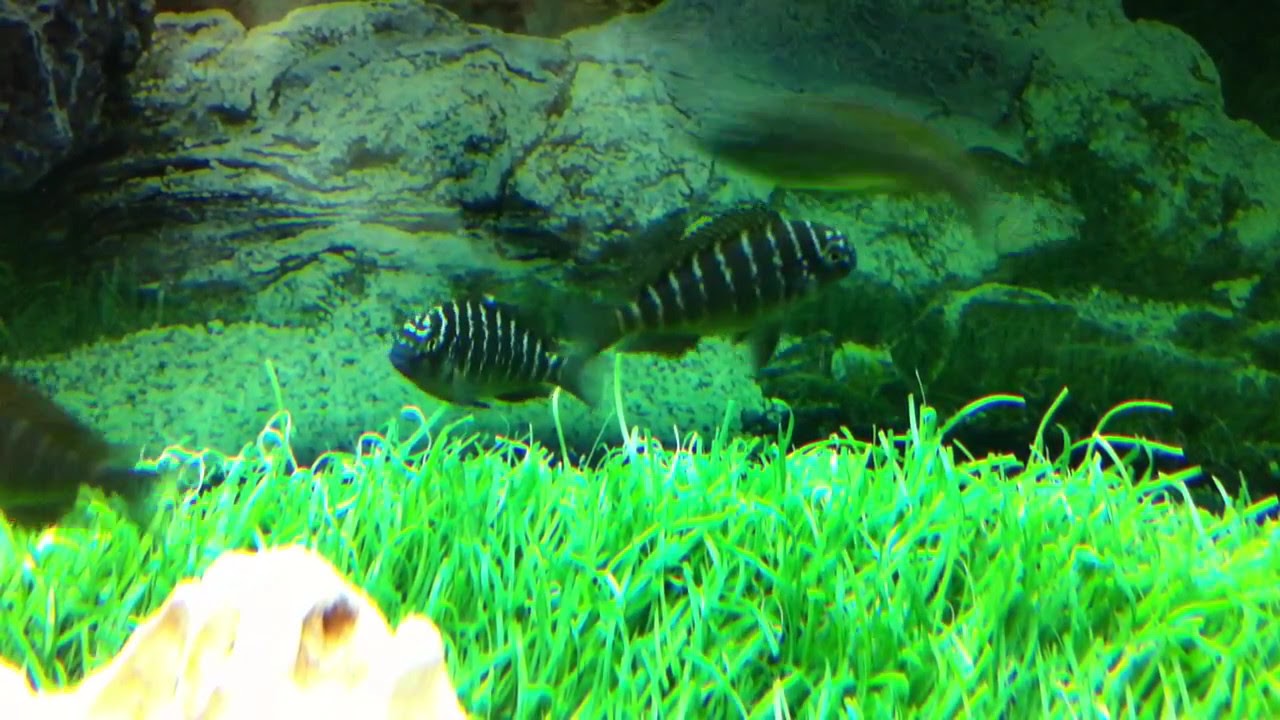This image captures a detailed scene inside a fish tank, focusing on two fish positioned centrally and oriented in opposite directions. Both fish are of the same species, characterized by their completely black bodies adorned with vertical white stripes, and they feature dark fins with small dark eyes. The bottom of the tank is covered with bright green sea grass that reflects light, creating striking highlights. In the background, there are rugged rock formations with a whitish texture that also contribute to the green-tinted hue that permeates the entire scene. The overall impression is that of an artificially lit, home or public aquarium rather than a natural aquatic environment.